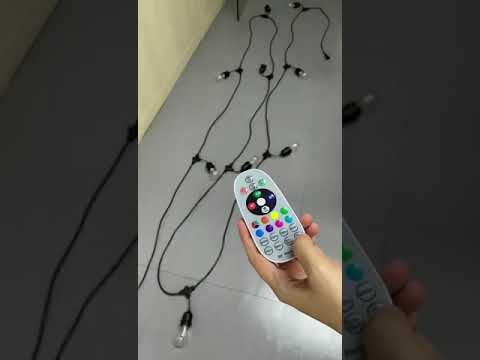The vertical cellphone-style image centers on a left hand holding a small, rounded remote control, extending from the bottom edge of the right side of the picture. The remote, which is grey and slightly tapered on one side, features a prominent black circular disc in the middle surrounded by numerous multicolored buttons including red, purple, green, blue, and teal. Some buttons bear unidentifiable words. Below this array, the controller rests above a shimmery, grey floor with a string of LED lights laid out, akin to large, clear Christmas tree bulbs. The background is creatively overlaid by a zoomed-in and faded version of the central image, enhancing the focus on the dazzling LED light controller in the hand.